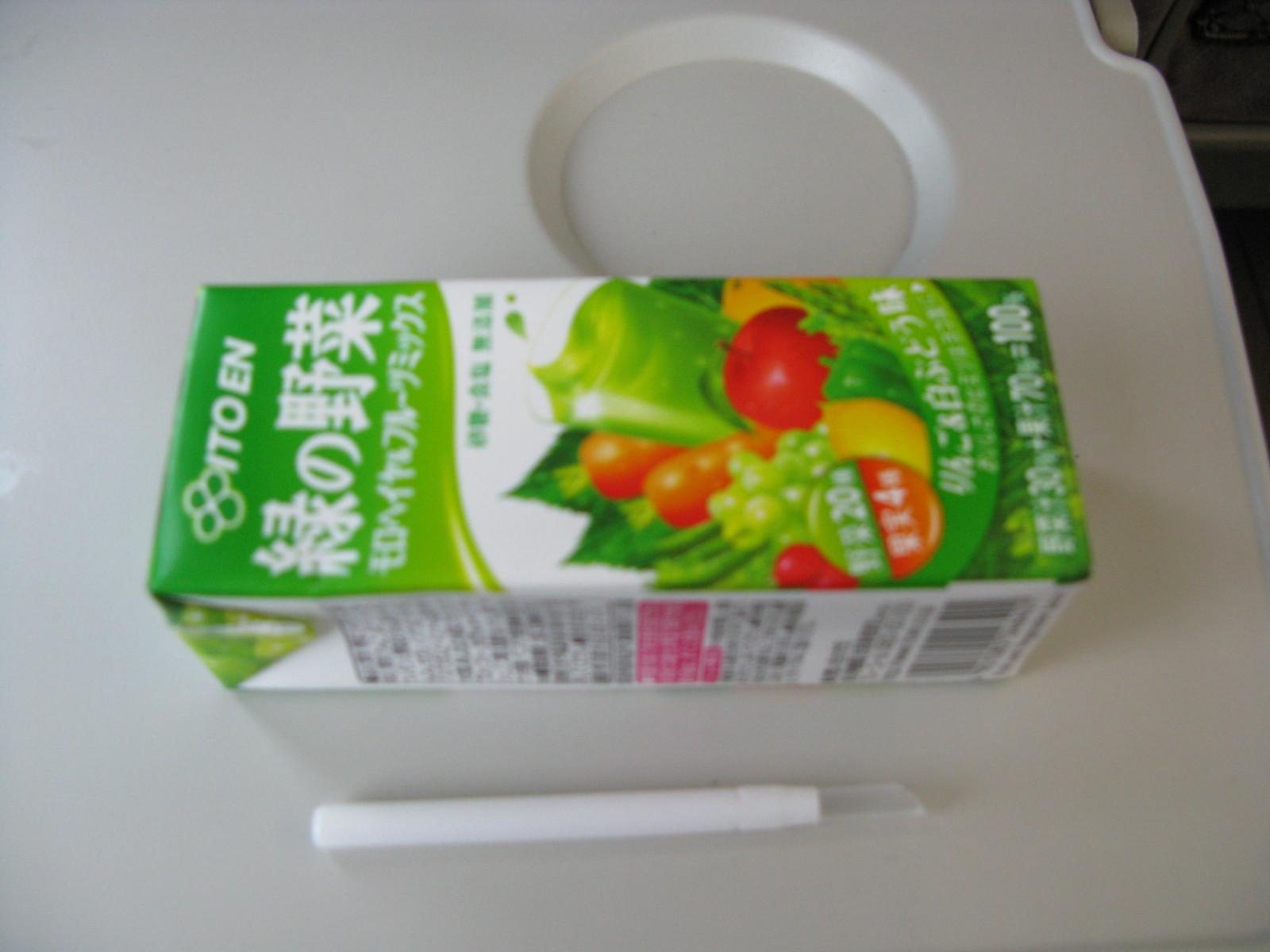The image is a color close-up photograph of a drink carton originating from Asia, as suggested by the predominantly Asian characters on the packaging. The carton, which contains juice or food, is lying sideways horizontally across what appears to be a greyish tray similar to those found on high chairs or airplanes. The top of the carton, which is green and features white writing, is oriented to the left, while the bottom of the carton is toward the right side of the tray. The carton showcases an assortment of produce on its front, including an apple, a green bell pepper, green grapes, carrots, possibly a lemon, and a glass of green juice. There are sections of the carton with white, pink, and black writing as well as a barcode near the bottom. A white straw with a clear, oblique pointy end, designed to pierce the carton for drinking, is placed on the tray below the carton. The tray itself has a circular recess for holding a cup, and a dark shadow appears in the upper right-hand corner of the image. Additionally, a small beige section peeks in from the upper right, possibly indicating another surface beneath the tray.